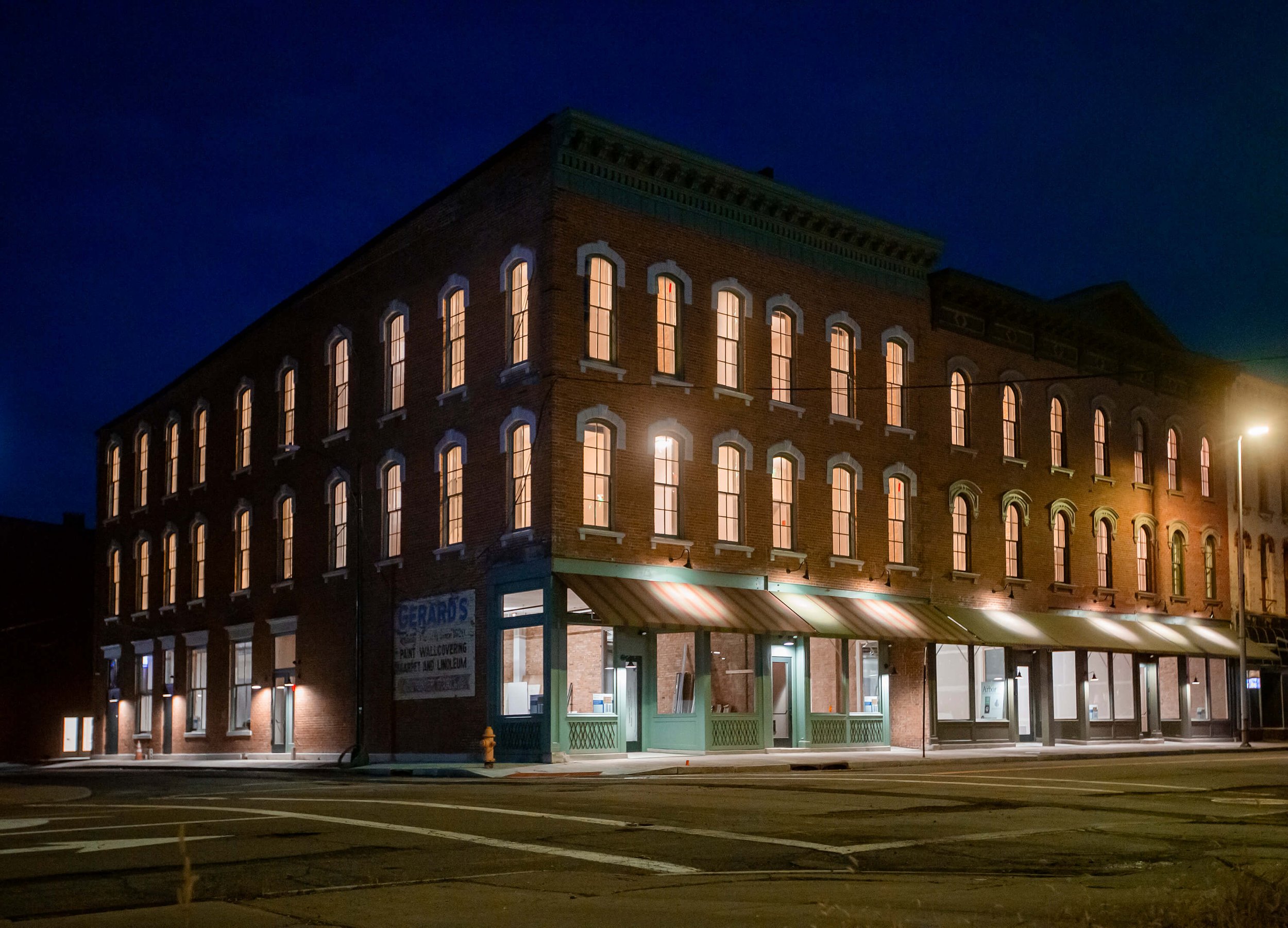The image features a historic, red brick building situated at the corner of a block, captured at nighttime. The structure, reminiscent of early 1900s architecture, is three stories tall with distinct vertical window panes. Illuminated warmly from within, the building’s numerous windows line the top and middle portions, casting a glow amidst the deep blue night sky. The building appears to be divided into sections, potentially for different shops or storefronts. The ground level showcases a mixed palette: on the right side, storefronts are decked with a green and yellow striped canopy, while sections on the left boast a brown trim around the windows. Prominently, a sign reads "Gerrard's" in blue on the left side. The scene is notably serene, with no people or cars visible, adding to the timeless feel of the photograph.